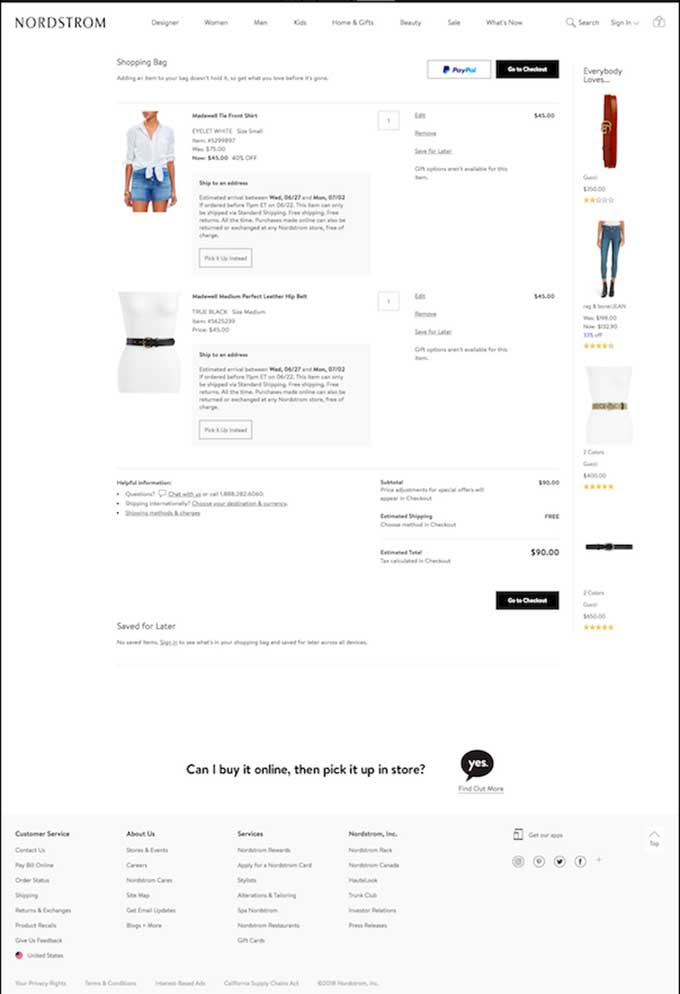This image is a detailed screenshot of the Nordstrom website interface. The webpage features a clean white background with predominantly black and gray text, accompanied by several images at the top of the page. On the left-hand side, the Nordstrom logo is prominently displayed in all capital letters. 

Across the top, a navigation bar contains eight category options, though the text is somewhat small and challenging to read. Adjacent to these categories, there is a search icon depicted as a magnifying glass, followed by a "Sign In" button and a shopping bag icon.

In the main section of the screen, the title "Shopping Bag" is prominently featured with a line of text beneath it. Next to this is a PayPal logo, accompanied by another button that has white text on a black background.

The right-hand side of the page showcases ads for different products, complete with prices, descriptions, and star ratings. There are four items listed: one pair of pants, a belt, another belt, and an indiscernible item.

Dominating the central part of the screen are two items displayed in the shopping bag. The top image features the torso of a woman clad in a white button-down shirt paired with denim shorts. The second image illustrates a black belt wrapped around a mannequin waist.